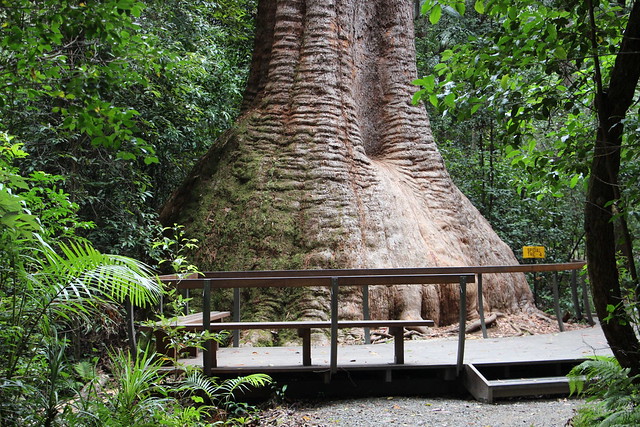This color photograph, taken during the daytime in a dense forest, focuses on an extraordinarily large tree with a massive trunk that resembles the foot of an elephant. The image captures the roots and moss-covered base of the tree, giving the impression that it has stood for centuries. Nestled amongst a variety of greenery including ferns and other plants, this humongous tree is surrounded by lush, overgrown vegetation. A gravel pathway leads up to a wooden platform with a bench where visitors can sit and admire the natural beauty. A yellow sign near the tree suggests guidelines, possibly indicating not to pass beyond the railing. The scene is enveloped in tranquility, offering a serene and almost enchanted forest atmosphere.